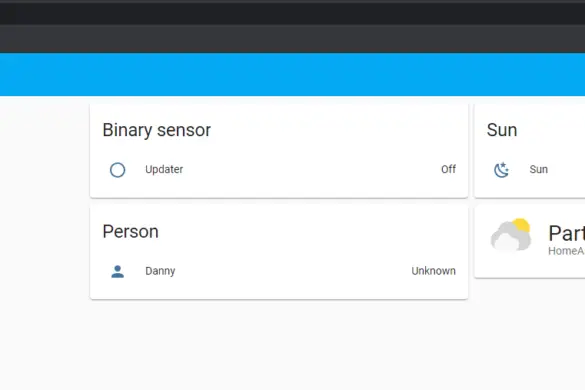The image appears to be a partial screenshot from an unidentified website, with no visible header, footer, or company name. The topmost part of the image features a narrow black border running horizontally across the width. Just below this black border is a dark gray section, followed by a strip of sky blue. The remainder of the background is white.

Centrally positioned in the image are the outlines of two rectangles in gray. The upper rectangle is labeled "Binary Sensor" in gray text. Below this label, it reads "Updater" with a gray circle to the left and the word "Off" to the right.

The lower rectangle displays the label "Person" and the name "Danny." To the left of this label is an icon resembling an account symbol: a small circle within a larger half-circle. To the right of "Danny," the word "unknown" is displayed.

To the right of these rectangles, there are two additional squares with white backgrounds and gray outlines. The top square reads "Sun" and, directly below in slightly smaller text, "The Sun." The icon inside this square appears more like a crescent moon than the sun.

Below this, in the white-background square, the partially visible text is "par," with the remainder cut off. Further below, another square shows the fragmentary labels "HOM" and a capital "A," with any additional text truncated. There is also an ambiguous gray half-circle with a yellow dot on its side, whose exact meaning is unclear.